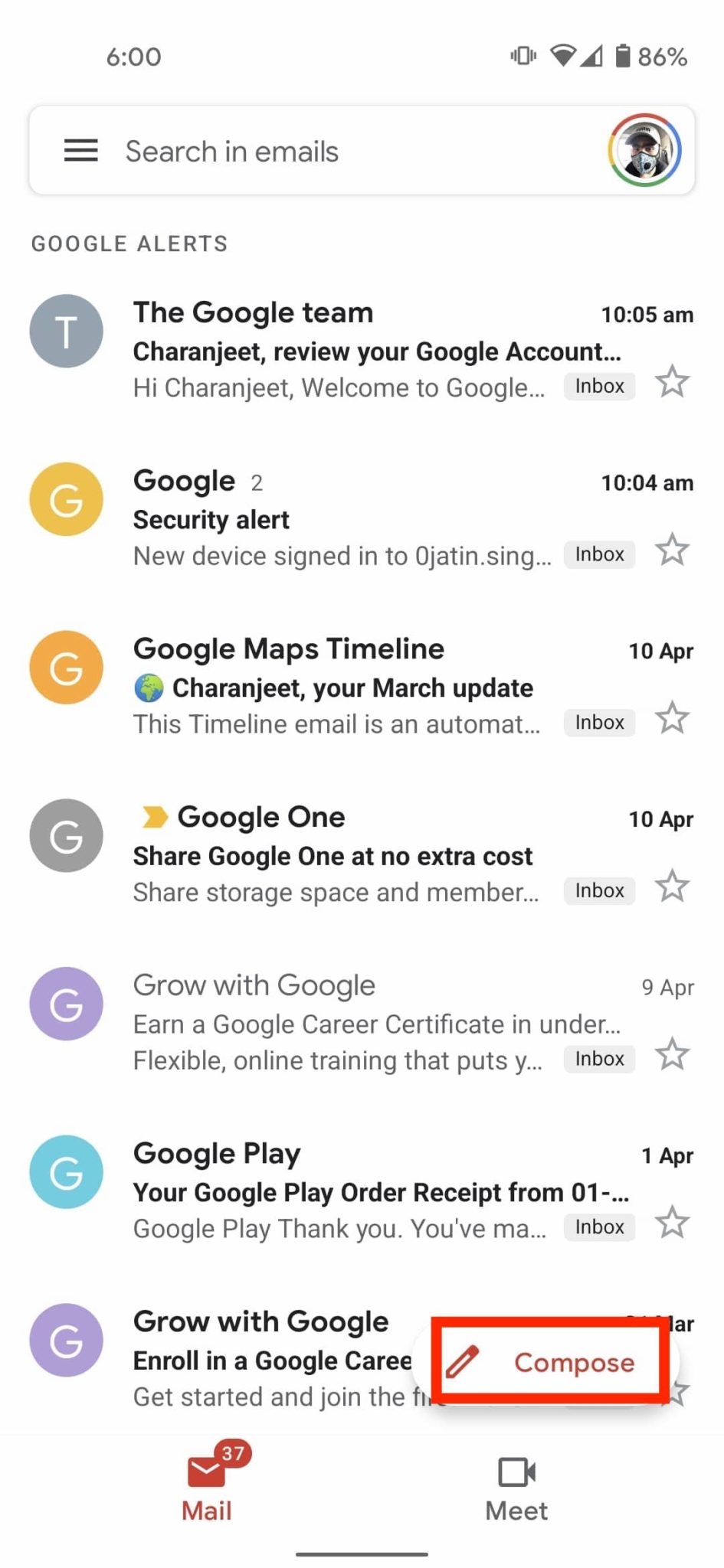This is a detailed screenshot of an email application on a smartphone. The top of the image displays the phone's status bar against an all-white background. On the left, it shows "6:00" in black, indicating the time. On the top right corner, the battery indicator shows 86%, mostly filled in black, followed by three full bars of both cellular signal and Wi-Fi, with the phone set to vibrate mode.

Below the status bar, a rectangular search bar spans the width of the screen. On the left of the bar are three horizontal black lines, stacked vertically. To their right, in black text, it reads "Search in emails." On the far right of the search bar is a colorful profile picture consisting of four quadrants: red at the top, blue on the right, green at the bottom, and yellow on the left, displaying an image of a man wearing a hat.

Under the search bar, in the left corner, the text "Google Alerts" is displayed. Below this, there is a small gray circle with a white "T" inside it and to the right, it says "The Google Team" in text, with the time displayed on the far right.

Next, in bold black text, is a header for the inbox items. To its right is a star icon. Following this, the first email preview shows two yellow circles with white "G"s, labeled "Google" and "Security alert," with the timestamp "10:04" on the far right.

The next email preview is from "Google Maps Timeline," dated "April 10." Beneath this, there are icons in varying colored circles: a gray circle with a white "G," a purple circle with a white "G," a blue circle with a white "G," and another purple circle with a white "G." Each entry continues with its respective header, a brief snippet of information, and timestamps on the right side.

At the bottom right, there's a red rectangle with a pencil icon outlined in red and the word "Compose" next to it. In the bottom left corner, a red email icon is present, with the number "37" written in white within a red circle above it, indicating unread messages. Below this, in red text, it says "Mail." On the opposite corner, there's an outlined black camera icon with the word "Meet" in black beneath it.